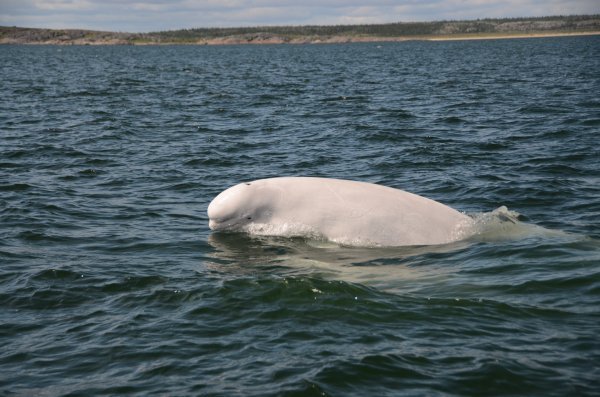This captivating color photograph features an ocean scene dominated by the deep, dark blue waters. At the center stage, a light gray beluga whale is breaching the surface, showcasing its head, eye, mouth, and blowhole with remarkable clarity. Positioned slightly to the left, the beluga appears to be looking towards the camera, with its tail and a small fin partially visible. The water surrounding the whale is calm with slight ripples, hinting at a gentle breeze.

In the distant background, the photograph captures a low-lying, flat coastline adorned with greenery and trees. A sandy beach and what seems to be an access road are faintly visible along the horizon, adding depth to the serene landscape. The sky above is mostly cloudy, casting a soft, diffused light over the entire scene. The overall composition exudes a sense of pristine tranquility, with the beluga whale being the undeniable focal point of the image.